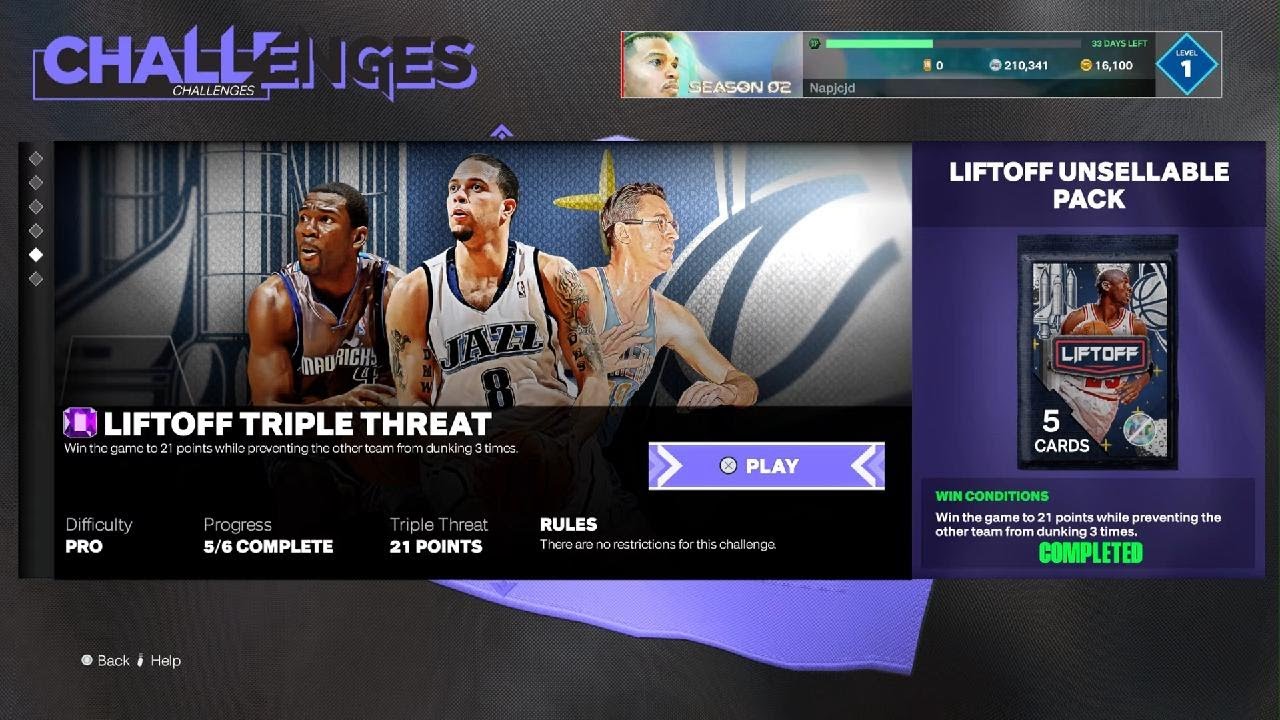This screenshot captures an in-game menu from an NBA-themed video game, possibly displayed on a computer monitor or TV screen. The dark-themed interface prominently features the word "Challenges" in a stylish purple and black font at the top left corner. Below this title, three NBA players are showcased in separate, adjacent photographs. The player on the far left is from the Mavericks, the middle player represents the Jazz, and the team of the player on the far right is not identifiable in this image.

Beneath these images lies the title "Lift Off Triple Threat," with smaller, unreadable text below it. An interactable "Play" button is positioned under this area, signifying that the user can start this specific challenge. Additional information indicates the "Difficulty: Pro," with the player's "Progress: 5 out of 6 Complete." The challenge involves a "Triple Threat" match, aiming for "21 points," though further rule details are too small to discern.

To the right of this challenge section, there's an image of a purchasable booster pack labeled "Lift Off Unsellable Pack." Accompanied by the term "Win Conditions," this virtual pack features five cards, collectively branded with "Lift Off," suggesting they offer some in-game advantage for completing the level.

In the top-right corner, the player’s stats are displayed, including their avatar and details about their progress in "Season 2," days remaining, current level, and virtual currency balance. This layout provides a comprehensive overview of the player's status and available challenges in the game.